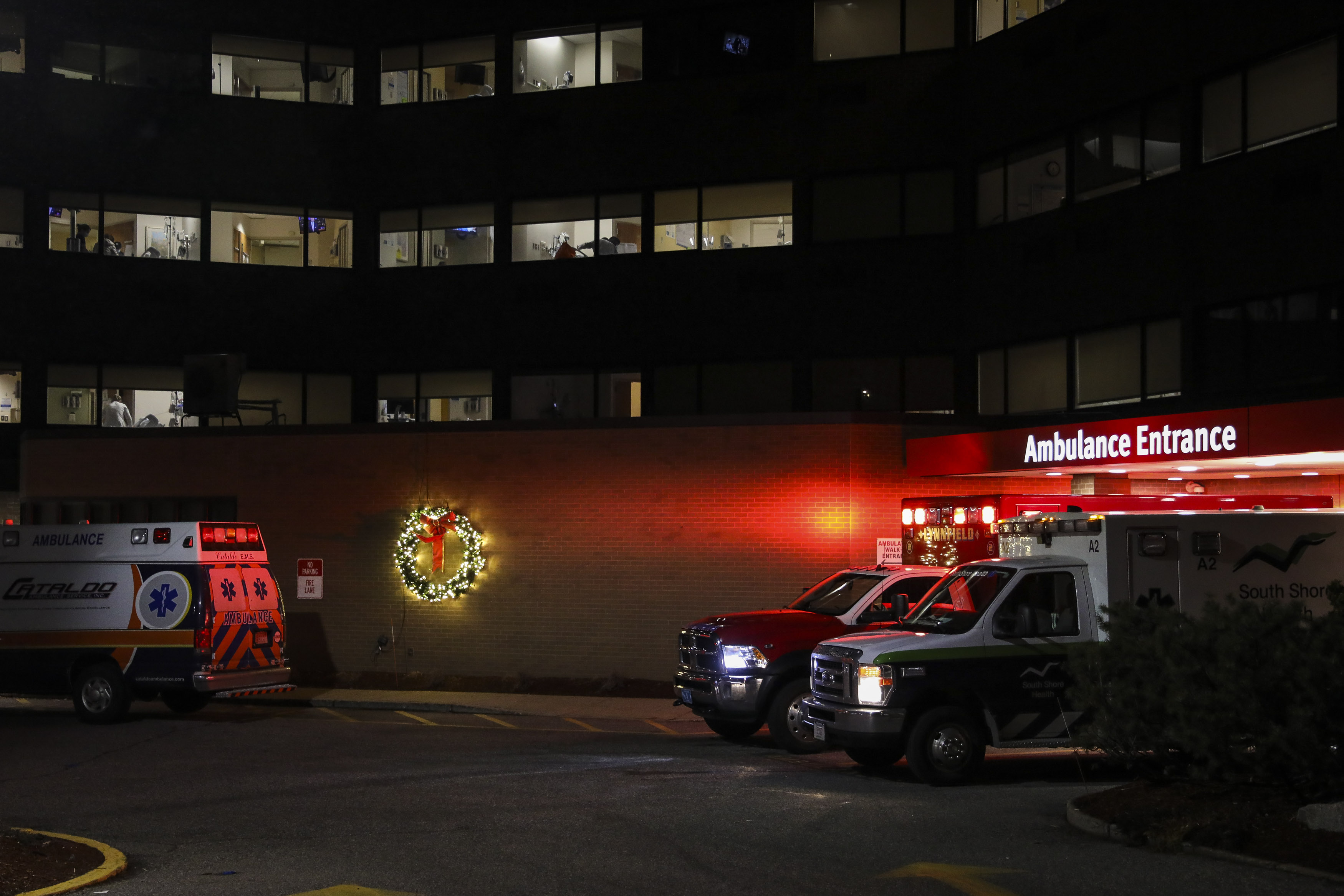The nighttime color photograph depicts a hospital's ambulance entrance, showcasing a dark scene illuminated by various lights. Prominently, a large Christmas wreath with a red ribbon and yellow lights decoratively hangs on a barrier wall beneath three stories of windowed hospital rooms. From some of these windows, warm, yellowish light filters through, while others are dark or obscured by drawn shades. Below the wreath, two ambulances are parked back-in under a covered area marked by a red sign reading "Ambulance Entrance." These two vehicles, one white and the other red, have their headlights on, casting a reddish glow onto the surrounding wall and vehicles. To the left, another ambulance, white with red and black trim, is positioned in the parking lot, facing the same direction as the backed-in ambulances, although its lights are off. The entire scene is framed by the hospital's brick facade and bathed in low ambient light, emphasizing the festive yet functional setting.